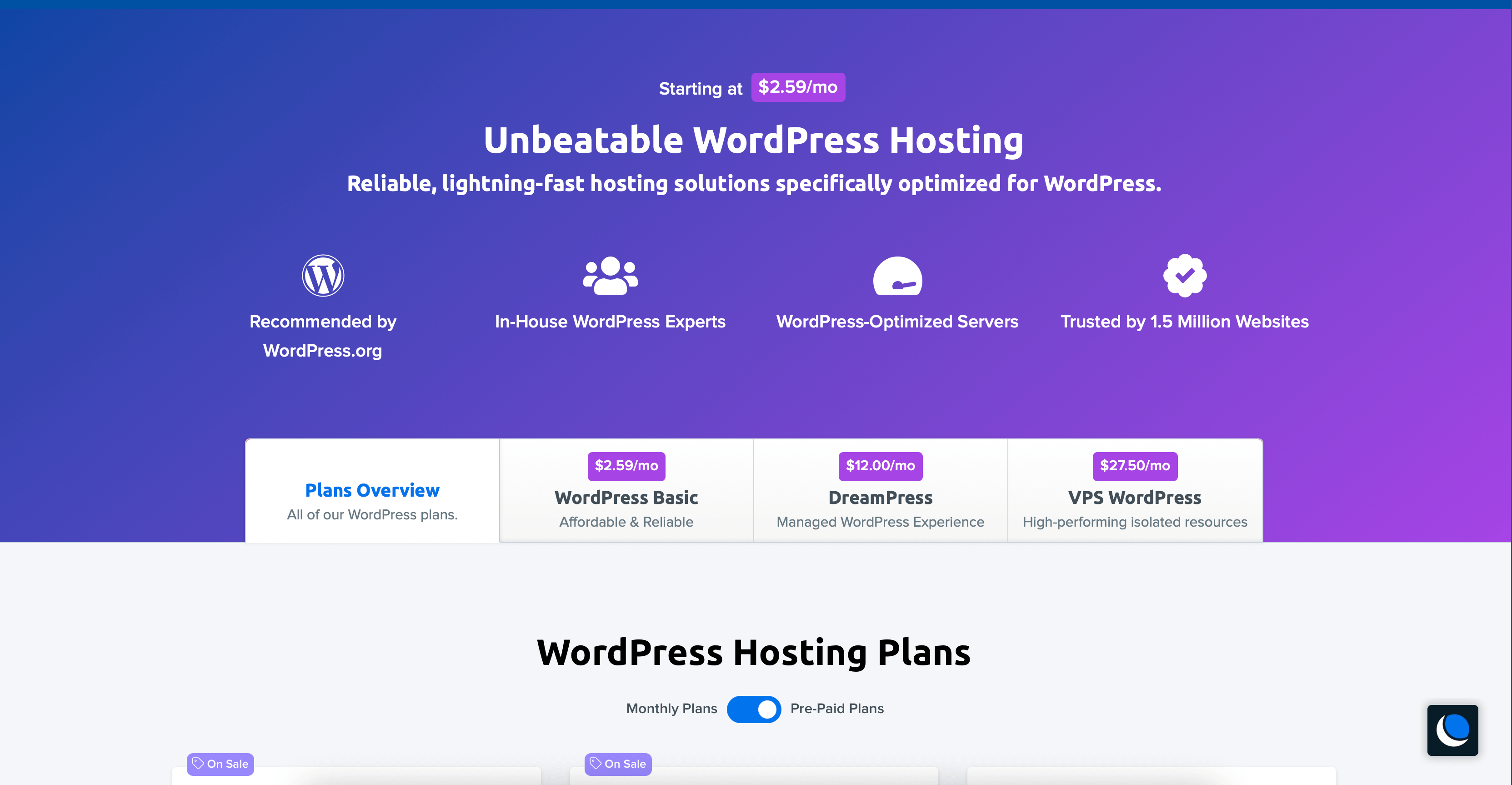The image captures a detailed view of a WordPress hosting page, showcasing various hosting plans and their features. 

---

At the very top, a bluish-purple gradient band stretches about two-thirds down the page, transitioning from blue on the left to purple on the right. Prominent white text reads "Starting at $2.59 per month," featured within small blue and purple boxes. The primary heading states "Unbeatable WordPress Hosting," advertising a "reliable, lightning-fast hosting solution specifically optimized for WordPress."

Directly below, an array of icons with accompanying text highlight key features of the service:

- A WordPress "W" icon with the text "Recommended by WordPress.org."
- An icon featuring three people with the label "In-house WordPress Experts."
- A speed dial icon next to the words "WordPress Optimized Servers."
- A tick box icon next to "Trusted by 1.5 million websites."

Beneath these icons, a whitish band extends across the page, with a slight gray tint noticeable towards the right side covering four panels. On the left, blue text announces "Plans Overview," followed by "All of our WordPress Plans." To the right, three distinct hosting plans are displayed:

1. **WordPress Basic:** Priced at $2.59 per month in a purple box, described as "Affordable and reliable."
2. **DreamPress:** Listed at $12 per month in a purple box, marketed as a "Managed WordPress Experience."
3. **VPS WordPress:** Costs $27.50 per month in a purple box, touted as a "High performance, isolated resource."

Below this section, another white band traverses the page horizontally with a central heading stating "WordPress Hosting Plans." Underneath, the text "Monthly Plans" is displayed alongside a blue slider set on "Pre-paid Plans." Small tags labeled "on sale" appear in the bottom left corner. More informational squares are visible, but the lower part of the image is cut off.

Finally, on the right side of the image, a distinct black square features a crescent moon icon. The moon, almost new, displays a white crescent with a blue surface forming part of a circle on its right, adding a contrasting element to the layout.

Overall, the image provides a comprehensive overview of the WordPress hosting offers, emphasizing affordability, reliability, and specialized performance.